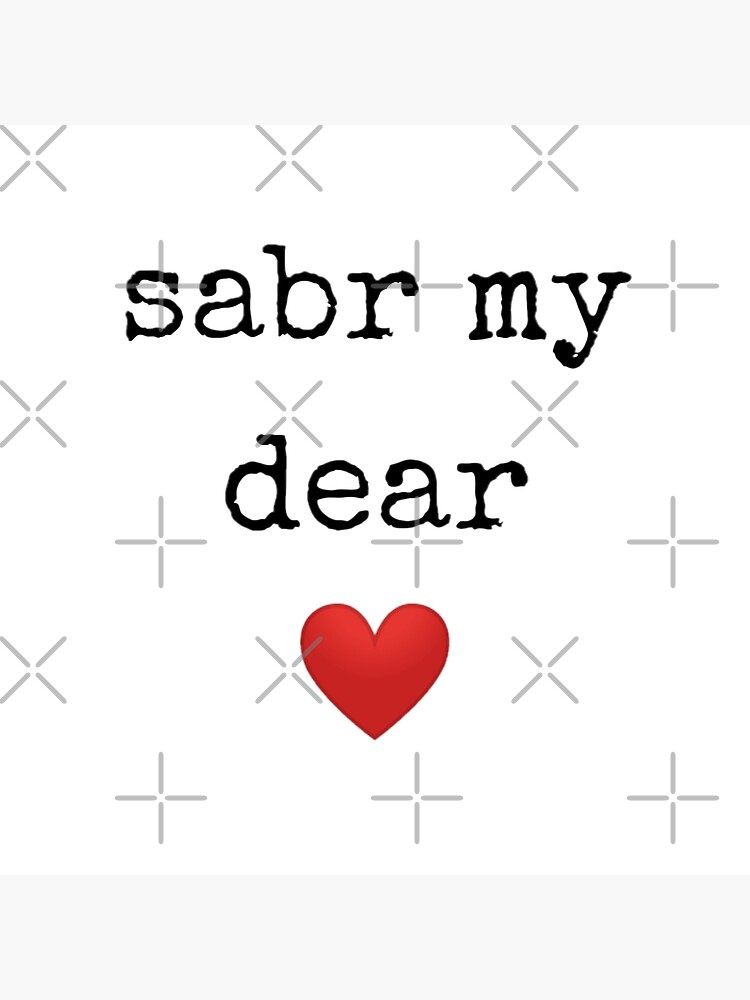The image is a stock photo intended for a greeting card, featuring the text "Saber, my dear" prominently displayed in the center. The text is rendered in chiller font, with "Saber, S-A-B-E-R, my" on one line and "dear" on the next line, followed by a simple, solid red heart outlined in a darker red color on the line below. The background is solid white, overlaid with a transparent pattern of alternating light gray Xs and plus signs arranged in four rows. The rows alternate in a consistent manner, creating a visually engaging backdrop that complements the central text and heart. There is no edging or border on the image, allowing the focus to remain on the affectionate message and its subtle, decorative background.